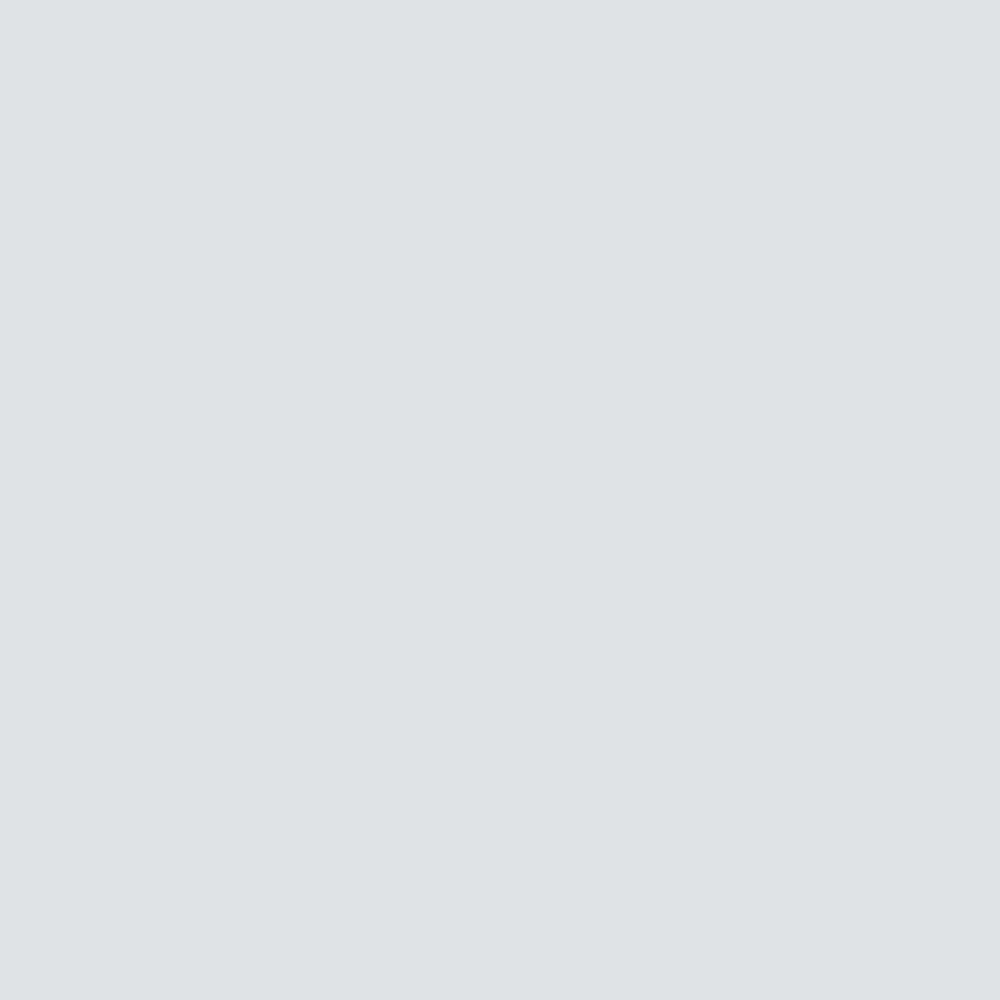A large, blank gray square occupies the center of the image, indicating a loading issue. The square, featuring four distinct corners, has a light gray background and contains no text, images, links, or icons. Above this square, a gray bar is visible, representing part of the webpage interface. This bar indicates task progress as "6 of 7 complete." To the right side of the screen, a yellow box prompts viewers with the message: "Think about what this image is at first glance." The entire scene underscores the absence of content, with the gray square serving as a visual placeholder for an image that failed to load.